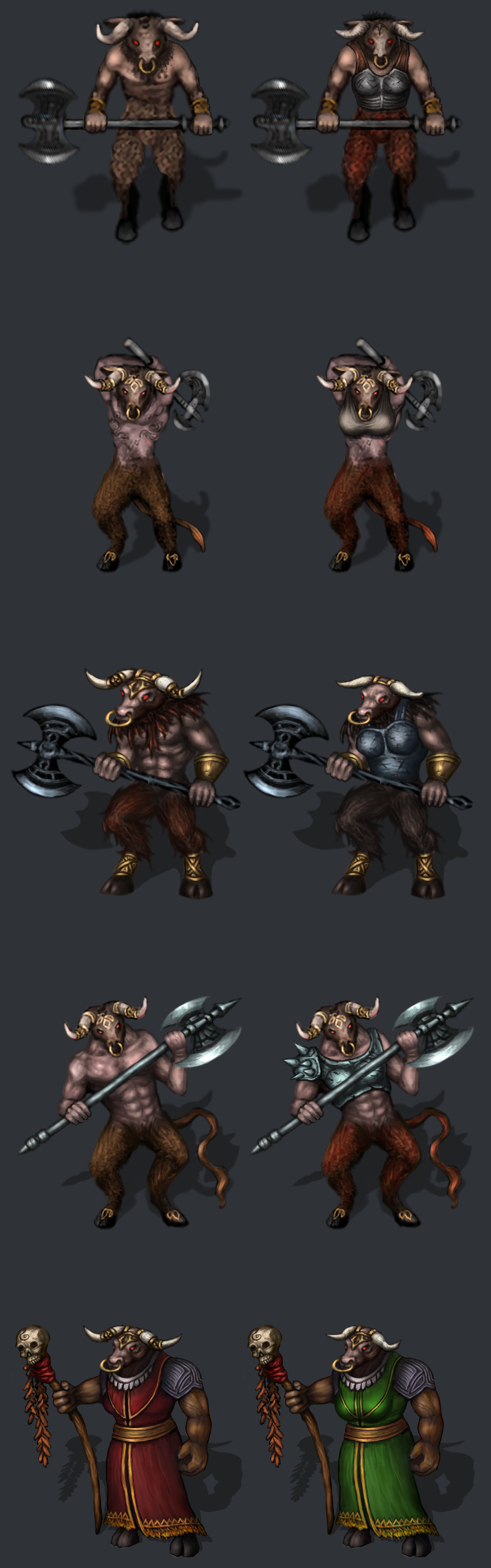The image features a series of anthropomorphic bull characters from the video game World of Warcraft. The layout is tall and narrow, organized into two columns of five rows each. The left column shows the male versions, and the right column shows the female versions, distinguished by emphasized breasts on the females. Each character is depicted in various poses, with a notable muscular build, red eyes, and a gold nose ring.

The topmost row portrays a humanoid bull wielding a two-bladed axe, depicted in various dynamic stances. Some poses show the axe held high as if ready to strike, while others have it held defensively in front. Different outfits adorn the character, ranging from shirtless to wearing partial or full body armor. Occasionally, more intricate details such as a tail are visible.

In contrast, the bottom row shifts from weapons to staffs topped with skulls, signifying a shift to more mystical or shamanistic roles. Correspondingly, the characters here are dressed in full robes—one red and one green—indicative of a priestly or magical nature. The consistent elements across all iterations are the anthropomorphic form, the prominent horns, and the detailed portrayal of various battle and priestly attire, exemplifying the versatile nature of this World of Warcraft character.